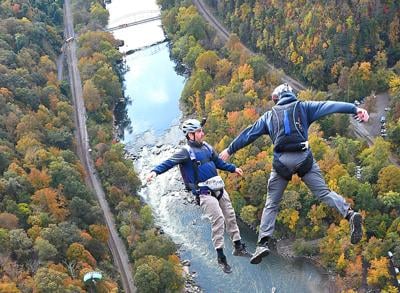The image captures a thrilling moment of two men bungee jumping from a significant height. The man on the left, wearing a blue shirt and beige pants, has a camera attached to his helmet. Both men are equipped with safety straps and helmets. They are suspended in mid-air above a picturesque autumn landscape, with a river flowing through the center of the scene. The river is flanked by trees adorned with a mix of orange, yellow, and green leaves, indicative of early fall. Above the river, a bridge is visible, with two roads running parallel to the riverbanks. The photograph, taken from an aerial perspective, provides a dynamic view of the men in freefall, emphasizing the beauty and exhilaration of the moment.